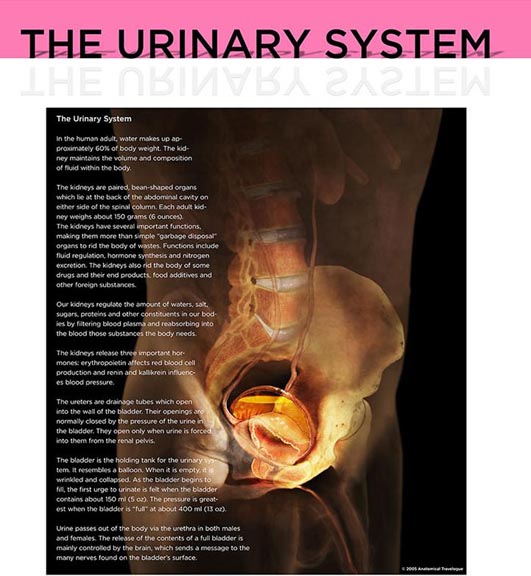The image is a full-color, rectangular medical poster with the title "The Urinary System" in black capital letters at the top, set against a dark background. The poster focuses on an illustration of the human urinary system, depicted in an X-ray-like format, highlighting visible parts of the lower body's anatomy including the spine, bones, urinary tract, and partially the reproductive organs. The poster's primary illumination accentuates the areas connected to the urinary system. Along the left-hand side, there are five paragraphs of descriptive text detailing the urinary system, written in small font, and a copyright notice dated 2004 is located in the lower right corner. The image appears to be educational in nature, designed to provide a detailed anatomical understanding of the urinary system.